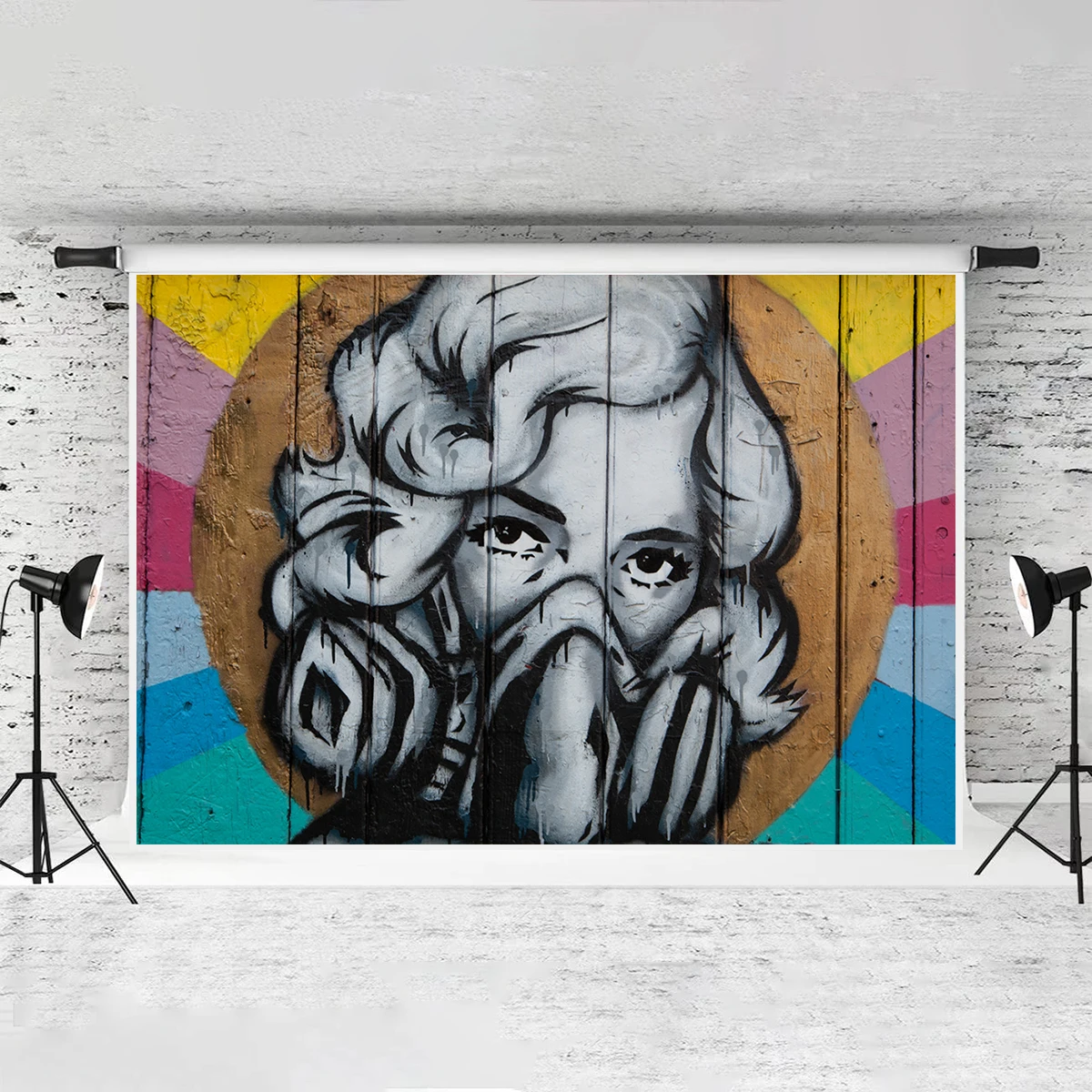The image features a large piece of artwork seemingly hung from the top of a white brick wall with areas of chipped away brown visible through the bricks. The wall also has some black lines faintly visible. The artwork itself appears to be a scroll or a large piece of canvas, rolled down and framed by black handles on each side. Depicted in the center of the canvas is a black-and-white image of a woman with short, curly, likely blonde hair and well-defined brown eyebrows. She is wearing a gas mask-like object covering her mouth and stares directly ahead. Surrounding her is a large brown circle, possibly resembling wood. Behind her, the background of the canvas features diagonal stripes in various bright colors including yellow, pink, fuchsia, lavender, light blue, aqua, and green. On both the left and right sides of the artwork, black tripods hold spotlights that illuminate the piece, emphasizing its intricate and surreal details.